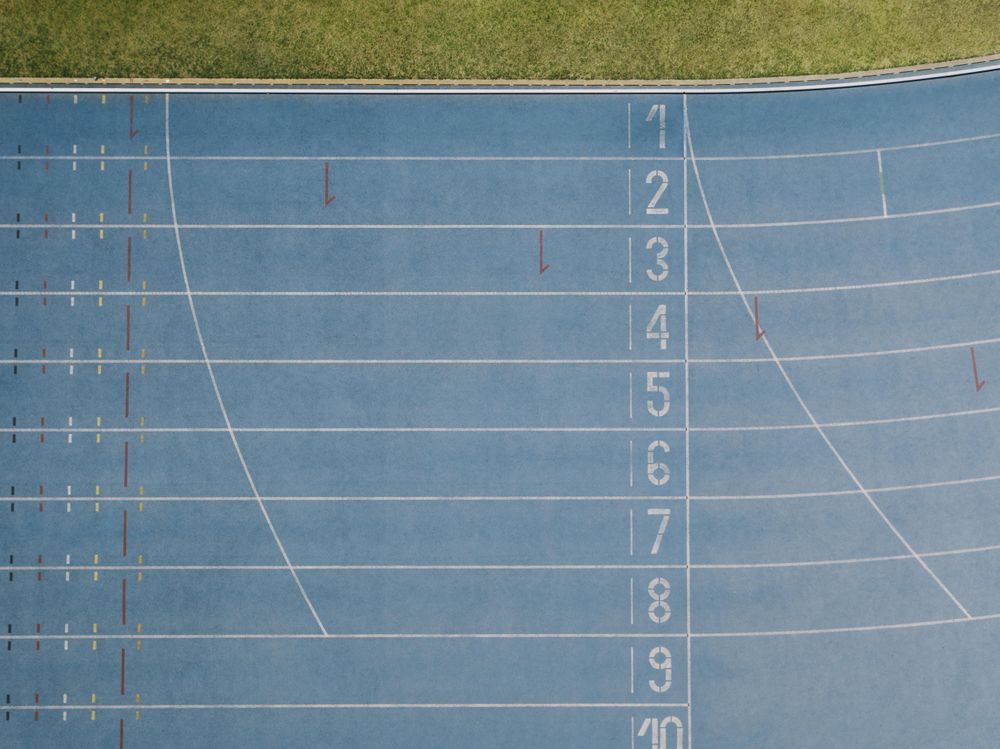The image depicts an aerial view of a worn, light blue running track surrounded by grass. The track features ten lanes, each clearly marked with white numbers from 1 to 10, running vertically down the middle of the track. Separating the lanes are horizontal white lines, while additional dotted white lines and one red dotted line add further detail. The track surface, slightly weathered, shows signs of extensive use. Curving gently towards the right are two identical, softly drawn lines, representing the beginning of the track bend. There are no signs or markings indicating the purpose or context of the track, but the image captures the tidy and well-maintained nature of the field and track.